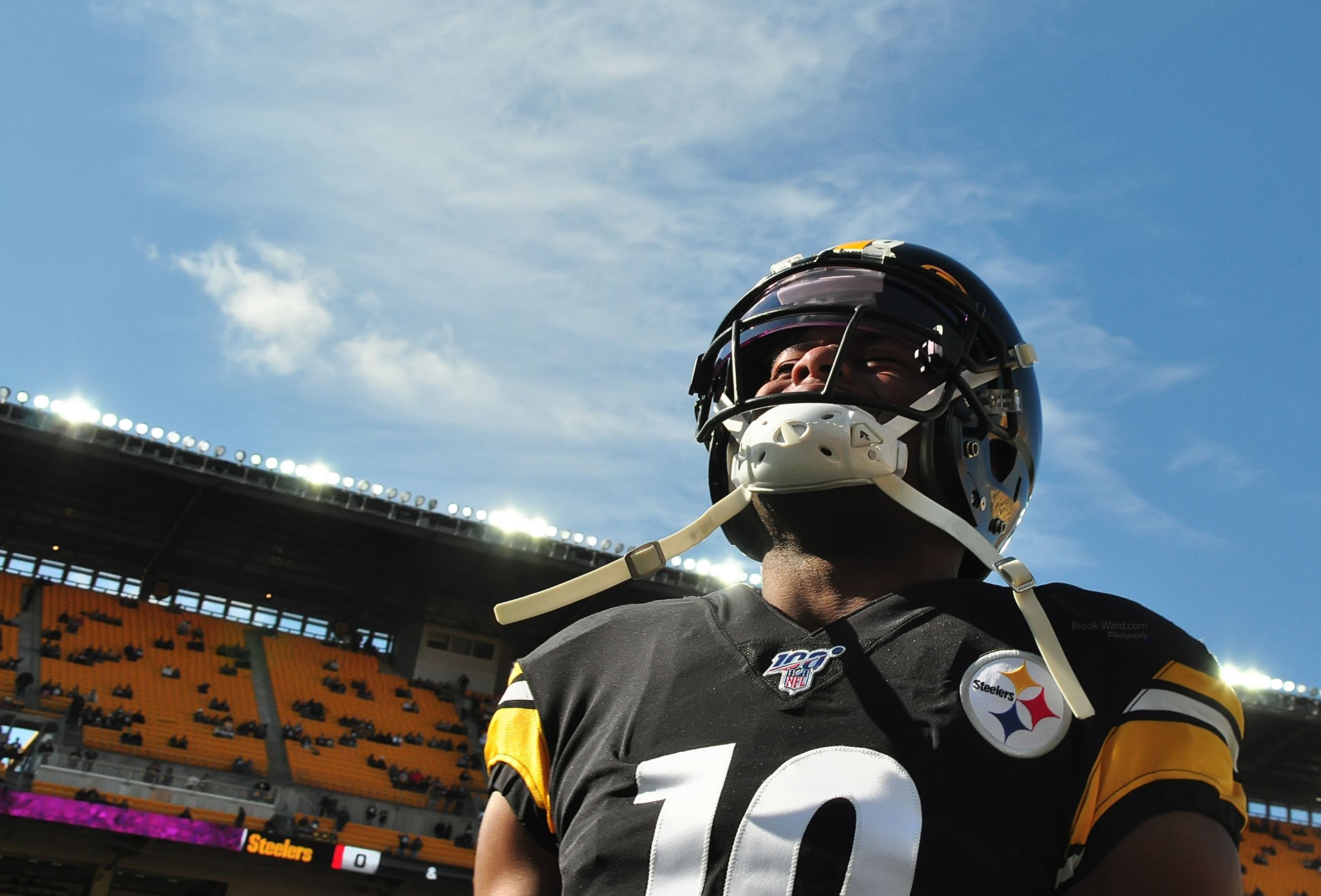This detailed photograph captures a close-up of a Pittsburgh Steelers football player, jersey number 10, on the field with the stadium in the background. The athlete, donning a black jersey with white "10" numerals and yellow short sleeves, stands under a bright blue sky with scattered, wispy clouds. The sun shines brightly on him, highlighting his black helmet and white chin strap, which dangles loosely. His gaze is directed upward as if anticipating the game ahead. The iconic Steelers logo, featuring yellow, red, and blue stars, is prominently displayed, along with the NFL 100 emblem on his uniform. The stadium lights are on despite the clear day, and behind him, only a few scattered spectators occupy the orange seats in the bleachers. The background elements, such as the partially filled stands and the stadium's roof, are subtly visible, adding depth to the scene without detracting from the player who remains the focal point of the photograph.